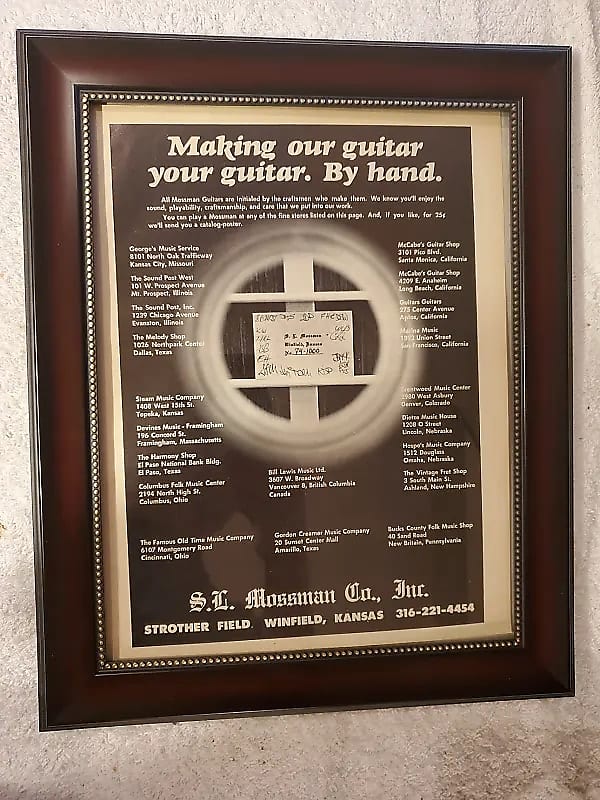This vertically aligned photograph showcases a dark brown, thick wooden frame adorned with gold dotted decor on its inner edge. The frame is mounted on a light tan stone wall, and inside it features a light gold matting. The centerpiece of the display is a poster with a dark brown background and cream-colored text at the top that reads, "Making our guitar your guitar by hand." In the middle is a white circular image that resembles a window, within which a note card, appearing like an index card, is centered. This note card seems to be positioned on an easel and contains handwritten, albeit illegible, text. Surrounding the circular image, there is more small white text aligned to the left and right, also too small to read clearly. At the bottom of the poster, in cursive, it says, "S.L. Mossman Co., Inc." Below this, in capital letters, the text states, "Strother Field, Winfield, Kansas, 316-221-4454." The image's primary focus is the intricate framed plaque, set against the contrasting texture of the stone wall background.